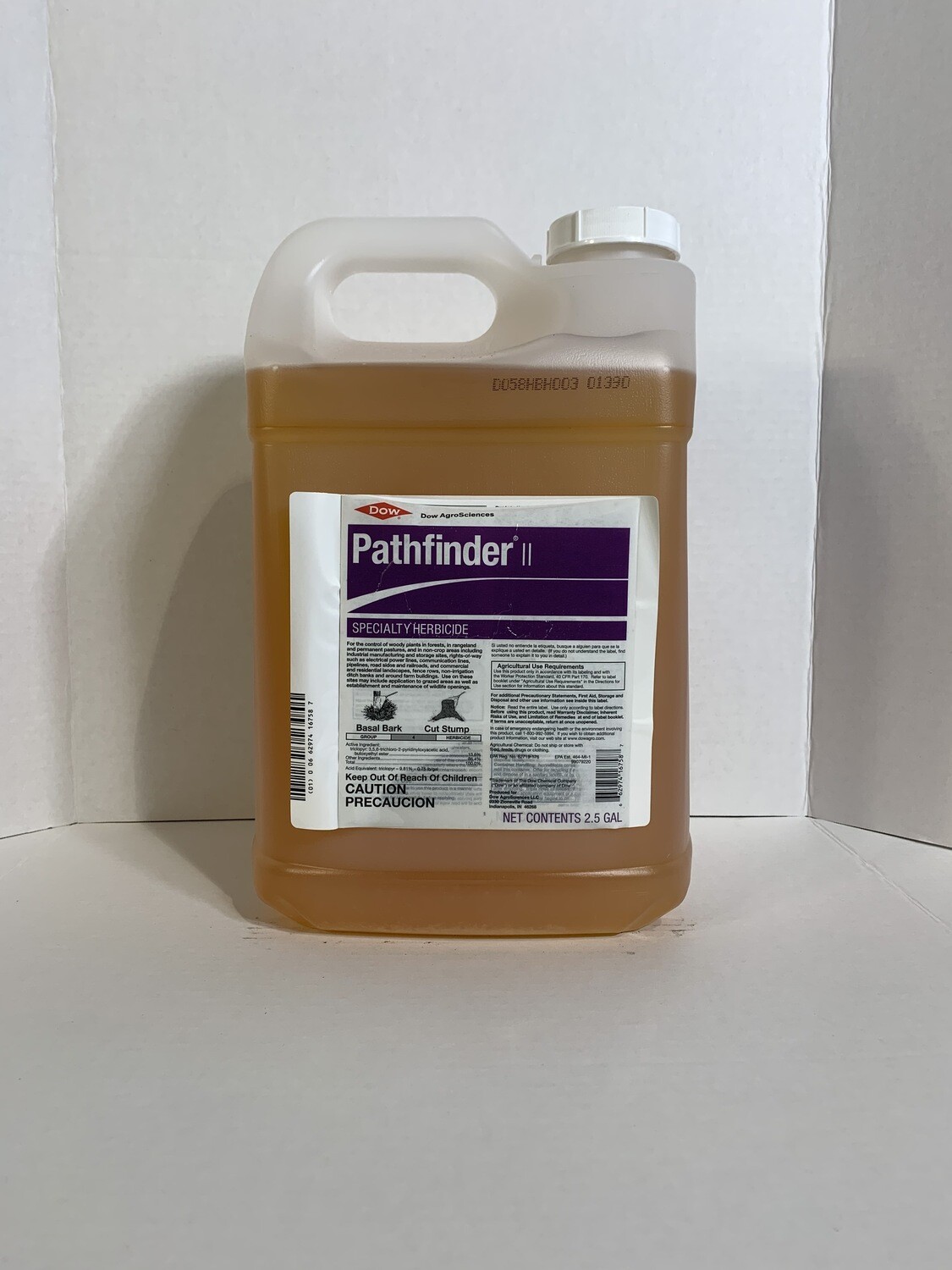The photograph captures a clear, rectangular, plastic jug with a handle at the top left and a large white cap at the top right, prominently placed on a plain white surface with a white backdrop. The jug, which holds a 2.5-gallon capacity, is almost completely filled with a yellowish-brown liquid. The label on the jug is white with a section of purple at the top and features a distinct red diamond logo with the word "Dow" written in white letters. "Pathfinder II Specialty Herbicide" is clearly printed on the label, alongside cautionary texts in both English and Spanish. The barcode is positioned on the left side of the label, and at the bottom right corner, the label states "net contents 2.5 gallons."